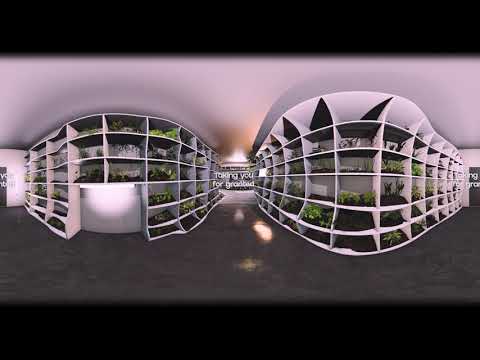The image depicts a computer-generated interior scene characterized by two towering walls of floor-to-ceiling cubbyhole shelving, each compartment meticulously housing various types of greenery. The shelves, structured in a grid-like pattern with approximately six levels, feature uniform brown dirt at the base and an array of verdant plants thriving above. A central corridor bisects the shelving units, creating a passageway that leads to a distant light, suggesting an entrance or door, though the details remain obscured. The floor, likely painted concrete, is a dark gray or black, contrasting with the stark white ceiling above. Although the writing in the center is blurred, it intriguingly reads "taking you for granted," adding a subtle, contemplative element to the otherwise botanical setting.